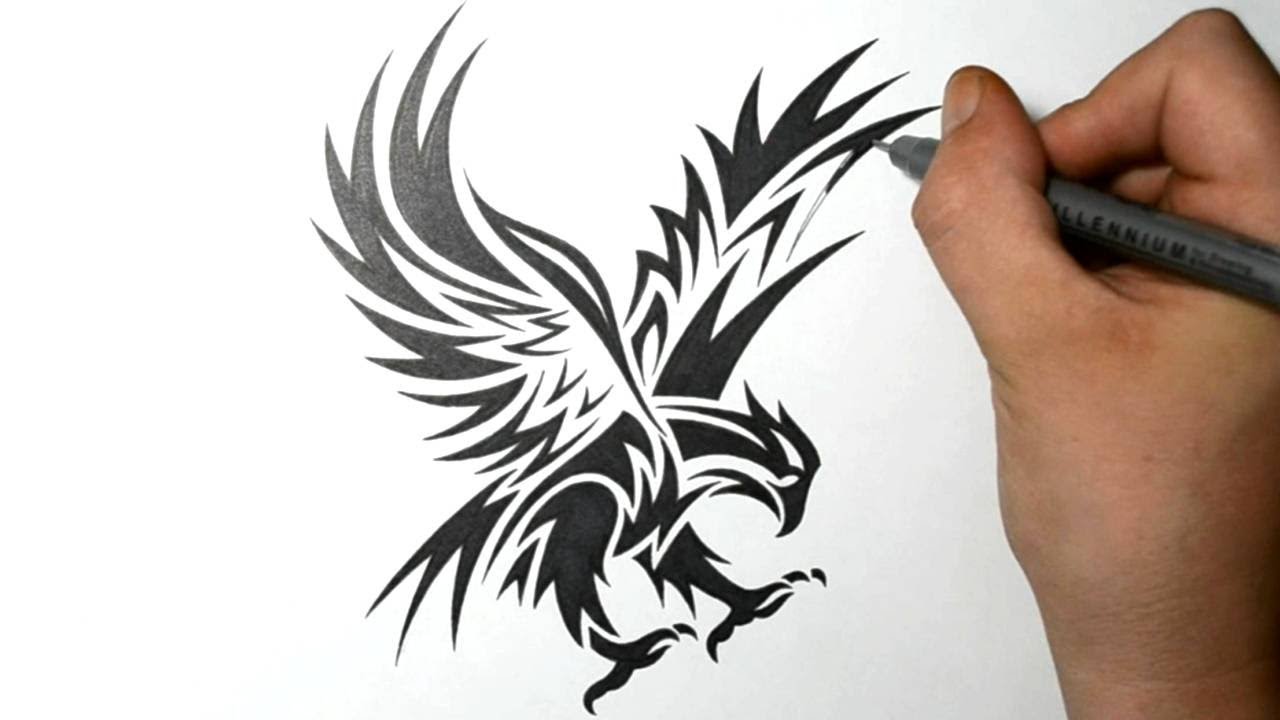The photograph captures a detailed, black ink drawing of a Phoenix or eagle-like bird with its wings outstretched, created on a white sheet of paper. On the right side of the image, there is a hand holding a fine-tipped, gray Millennium ink pen, actively adding intricate details to the drawing. The bird, with strong black outlines, showcases a tattoo-style appearance, featuring three distinct layers of feathers, a defined head and beak, and sharp black talons below. The artistic technique employs high contrast, highlighting different layers of feathers by leaving certain sections white, enhancing the visual depth. The bird appears to be poised mid-flight, perhaps about to land. The drawer's hand, likely a man's based on the short, unpolished nails, is in the final stages of perfecting the wings, emphasizing the realism and stylized elegance of the artwork.